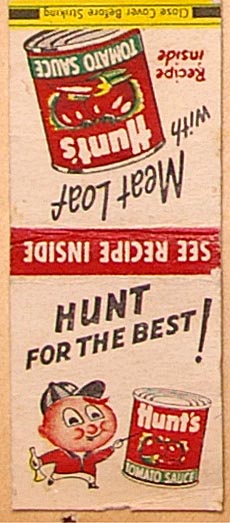This is a photo capturing an advertisement on a matchbook. The matchbook, which is laying flat, is positioned on a piece of peach-colored paper. The cover of the matchbook is upside down, also laying flat, set against a contrasting white background. The top of the cover prominently features the word “MEATLOAF” in bold black letters, followed by the word “WITH” and an image of a Hunt’s tomato sauce can directly beneath it. Towards the bottom left corner, the text “RECIPES INSIDE” appears in vibrant red. Spanning the bottom edge is a yellow banner with the instruction “CLOSE COVER BEFORE STRIKING” written in black text. The spine of the matchbook is highlighted with a red banner that states "SEE RECIPE INSIDE" in white letters. On the back cover, the slogan “HUNT FOR THE BEST” is printed alongside an illustration of a little round boy wearing a striped hat. The boy is pointing at an image of a Hunt’s tomato sauce can with his right hand while holding a trumpet in his left hand.